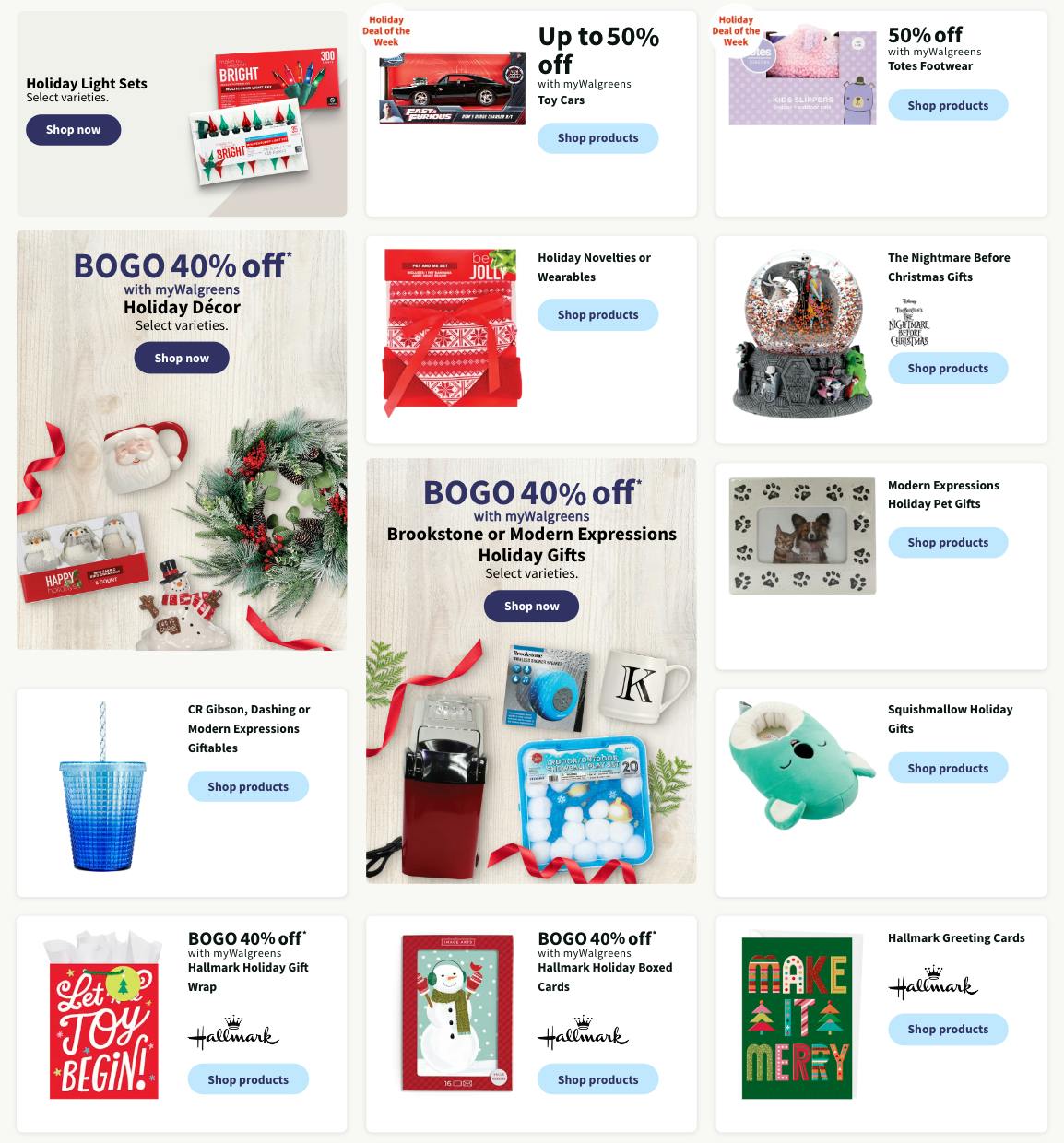The image depicts a small, somewhat blurry advertisement featuring various holiday-themed products on sale at Walgreens. In the top left corner, there's a message about a "Holiday Light Set" available in select varieties, with a dark blue button labeled "Shop Now." The promotion offers a "Buy One, Get One 40% Off" deal for holiday decor with a Walgreen's membership.

The image also showcases several Christmas ornaments, a snowman, a Santa Claus-themed coffee mug, and a wreath adorned with red ribbons. Below this, there's a section about "C.R. Gibson Modern Expressions," encouraging shoppers to "Shop Products," with a similar "Buy One, Get One 40% Off" offer.

Additionally, the ad highlights Hallmark holiday gift wrap with the cheerful message "Let Joy Begin." To the right, there's information about another promotion stating "Buy One, Get One 40% Off" applicable to Breakstone or Modern Expressions holiday gifts, again with a prompt to "Shop Now."